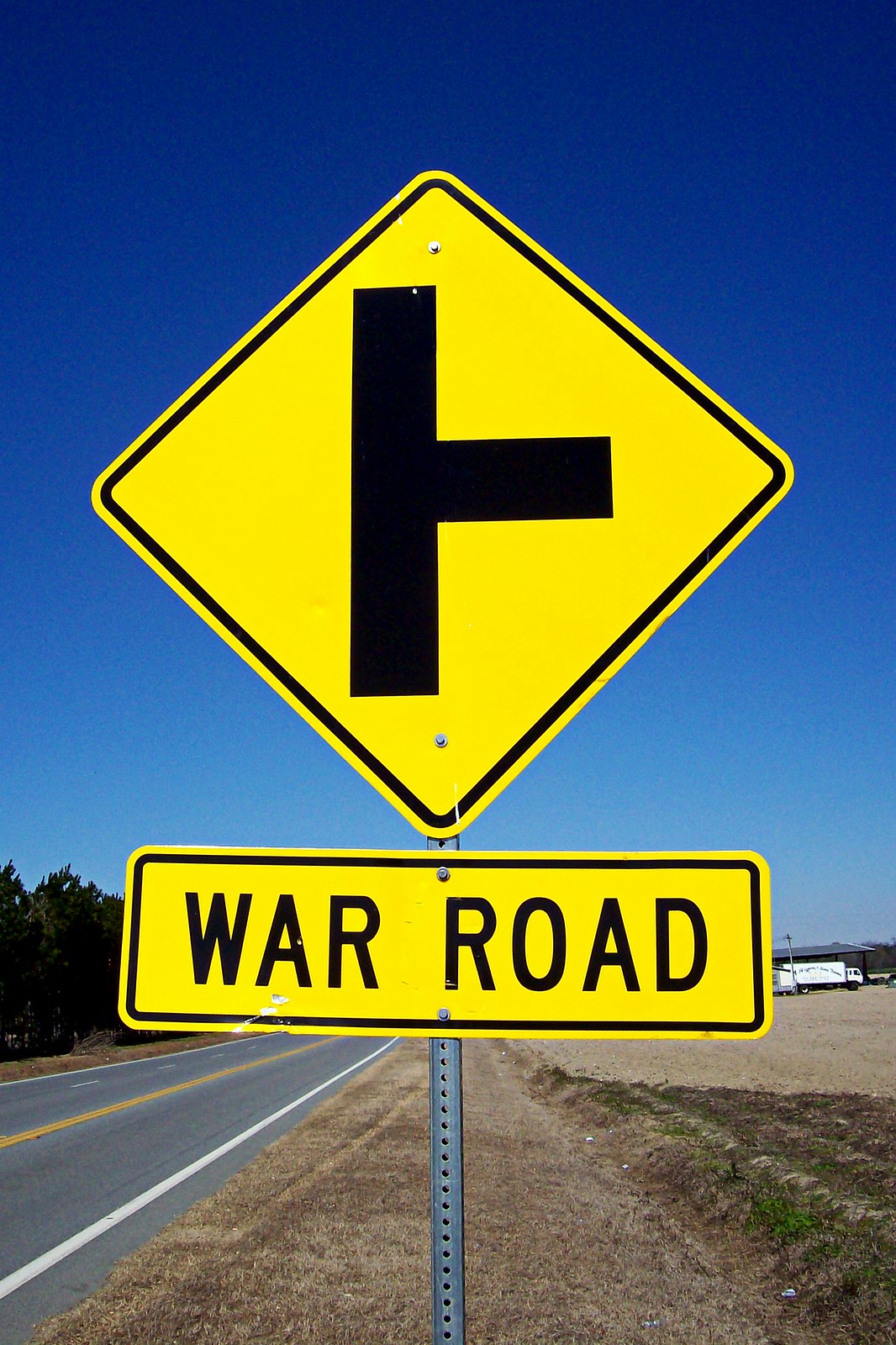This high-resolution photograph, oriented in portrait mode, captures a tranquil scene on a bright, sunny day. The sky above is a vivid blue, providing a cheerful backdrop for the roadside view. On the left-hand side of the image, a two-lane gray road stretches into the distance, marked by a prominent yellow stripe down the middle. Lining the road are lush green trees, their leaves rustling gently in the breeze.

Positioned on the roadside is a significant road sign. The upper portion of the sign is a yellow diamond, signaling the end of a road with a clear black marking. Beneath the diamond, a rectangular yellow sign is displayed, bearing the black text "War Road." The roadside itself appears dry and parched, featuring patches of dead, brown grass. This juxtaposition of the vivid sky, the well-maintained road, and the arid roadside creates a strikingly detailed and evocative scene.